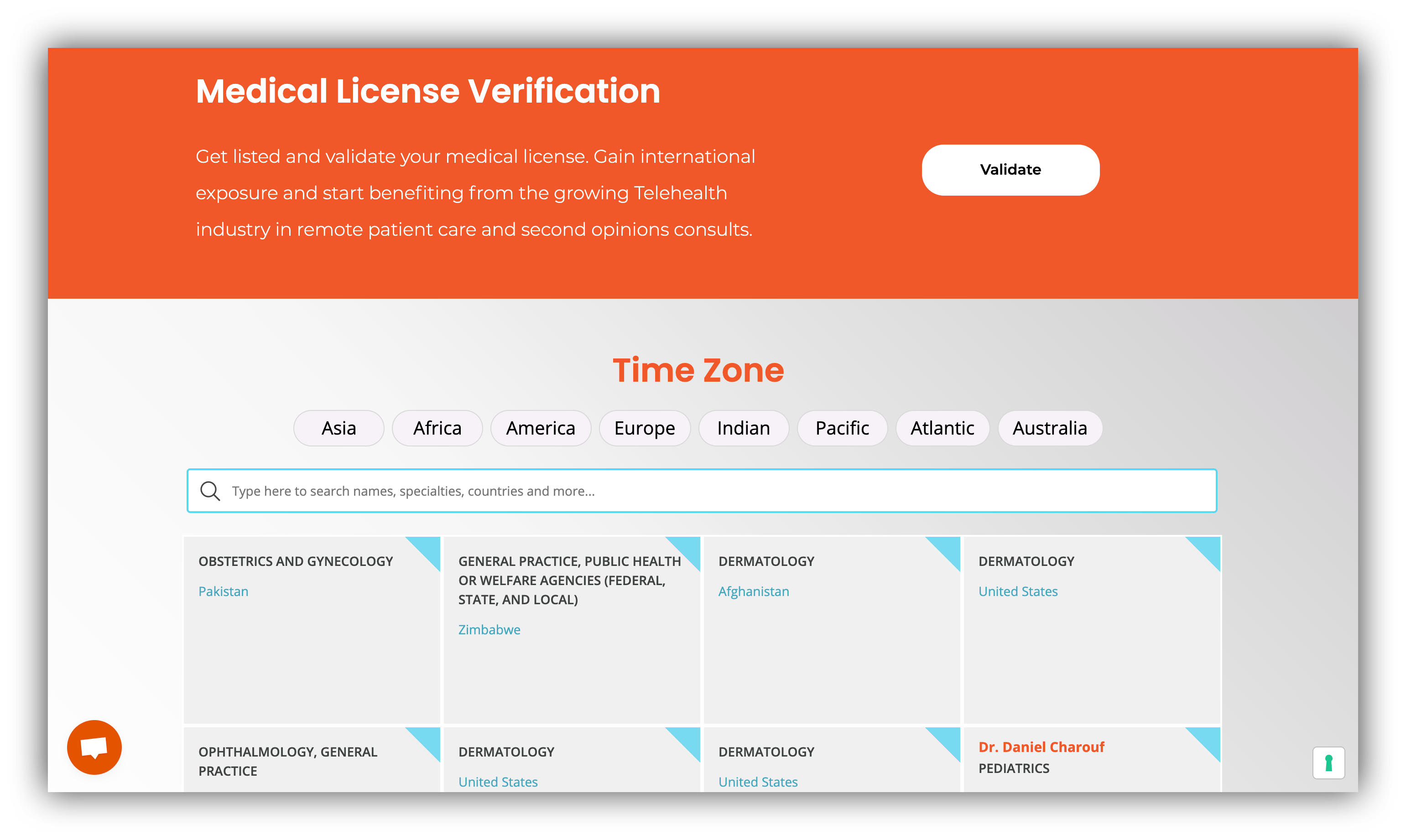A comprehensive and user-friendly computer pop-up screen titled "Medical License Verification" is displayed, aimed at medical professionals. The interface encourages users to "Get listed and validate your medical license" to gain international exposure and benefit from the rapidly growing telehealth industry, particularly in remote patient care and second opinion consultations. A prominent white "Validate" button is available for quick action. Below, various time zones are listed, including regions like Asia, Africa, America, Europe, Indian, Pacific, Atlantic, and Australia, facilitating global participation. Additionally, there are multiple checkboxes for different medical specialties such as Obstetrics and Gynecology, General Practice, Public Health, and Dermatology. Further options are available by scrolling down.